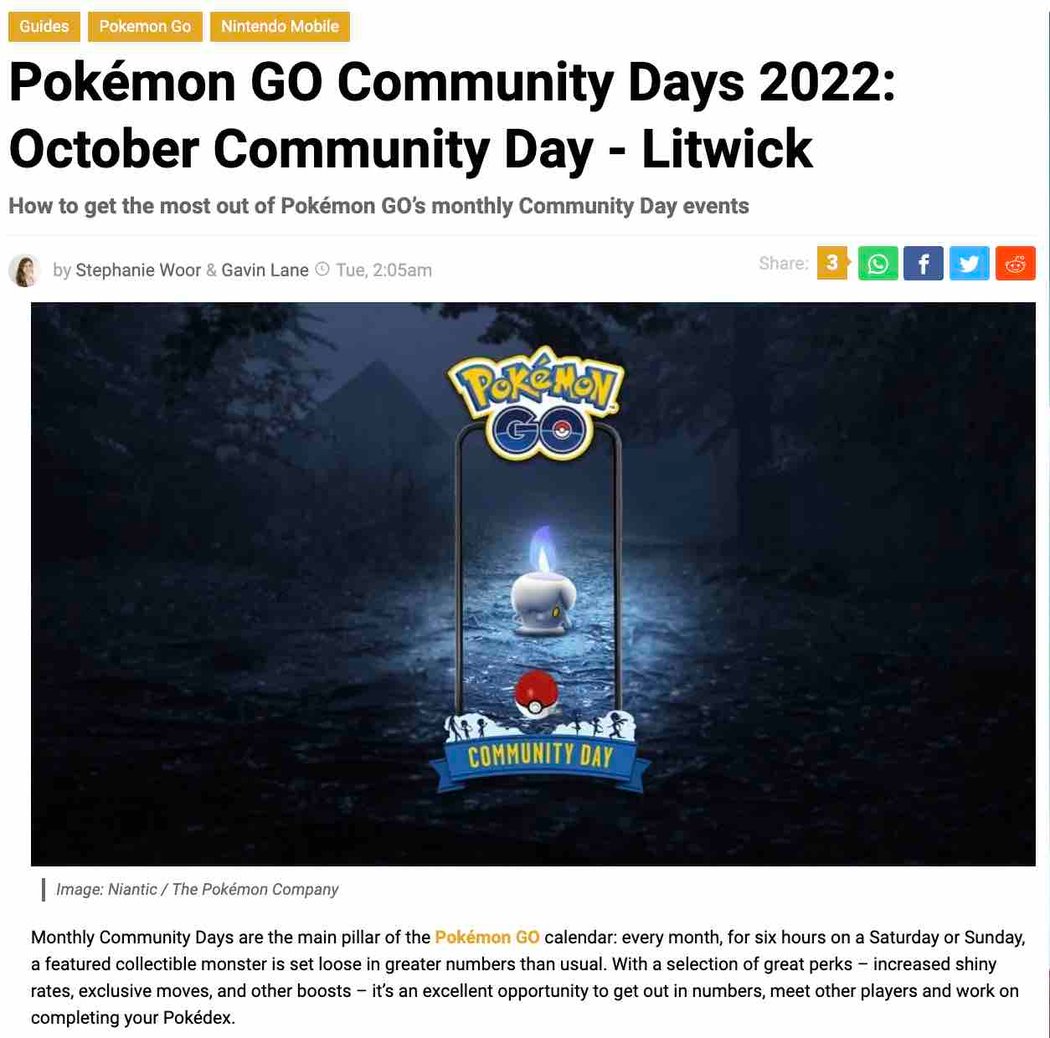The image is a screenshot from a website dedicated to Pokémon Go, specifically discussing Community Days for 2022. The webpage appears under the section "Guides" and is titled "Pokémon Go Community Days 2022" with a focus on the "October Community Day: Litwick." Authored by Stephanie Woor and Gavin Lane, the article was published at 2:05 a.m. The image credits are attributed to Niantic and The Pokémon Company.

Community Days are described as a key feature of the Pokémon Go calendar, taking place for six hours on selected Saturdays or Sundays each month. During these events, a featured collectible Pokémon appears in greater numbers than usual, alongside perks like increased shiny rates, exclusive moves, and other benefits. These events encourage players to socialize, collaborate, and progress towards completing their Pokédex.

At the center of the screenshot, there is an image prominently displaying the Pokémon Go logo, featuring the iconic red, white, and black Pokéball. The overall layout is rectangular, with the photograph breaking up the text-heavy content. Other than the logo, the photograph is simple, serving more as a branding element than a focal point.